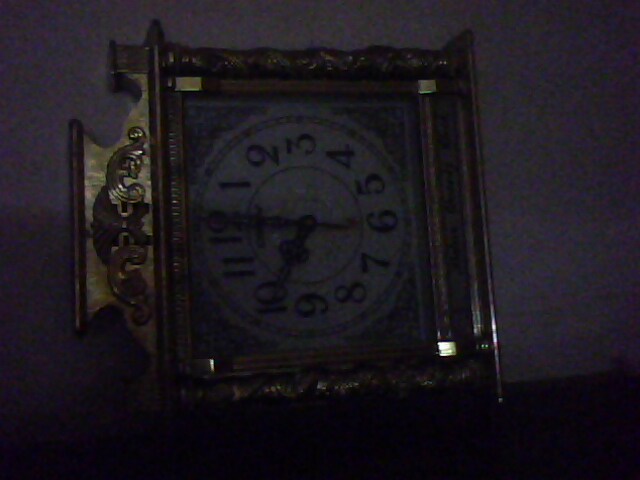This image features a clock that appears to be oriented horizontally, though it is typically intended to be displayed vertically. The clock face, which is adorned with the numbers 1 through 12, is positioned on its side with a central white circle indicating the clock’s center. Radiating from the center are ornate, patterned hands marking the time. The clock face is encircled by an intricate bluish or blackish pattern, particularly noticeable in the corners. Surrounding the clock face is a gold-colored border filled with elaborate designs, adding to the clock's opulent appearance. The room in which the clock is displayed is quite dim, with shadows casting over the clock, obscuring some details. The clock hangs on a whitish wall, and a notable black spot is seen near the bottom of the image.